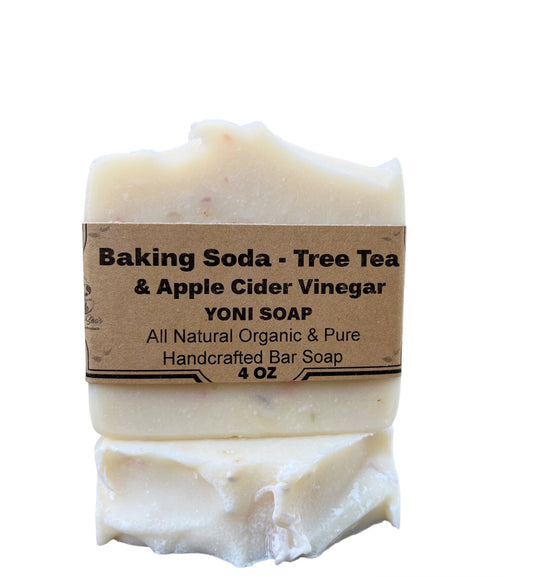In the image, there's a handcrafted bar of soap with an irregular shape, predominantly featuring an off-white or beige-y tint. The soap contains various specks and flakes, including tan, black, orange, red, green, and possibly purple, suggesting natural ingredients like tree tea leaves or bits from apple cider vinegar. The bar is perched on a broken piece of soap of similar color, emphasizing its artisanal nature. Encircling the soap is a simple, rustic brown paper band resembling a paper sack, adorned with black writing. The label reads: "Baking Soda, Tree Tea, and Apple Cider Vinegar," followed by "Yoni Soap." In smaller font, it declares, "All-Natural, Organic, and Pure, Handcrafted Bar Soap," and indicates that it weighs four ounces. The overall presentation exudes a sense of natural, handmade quality.